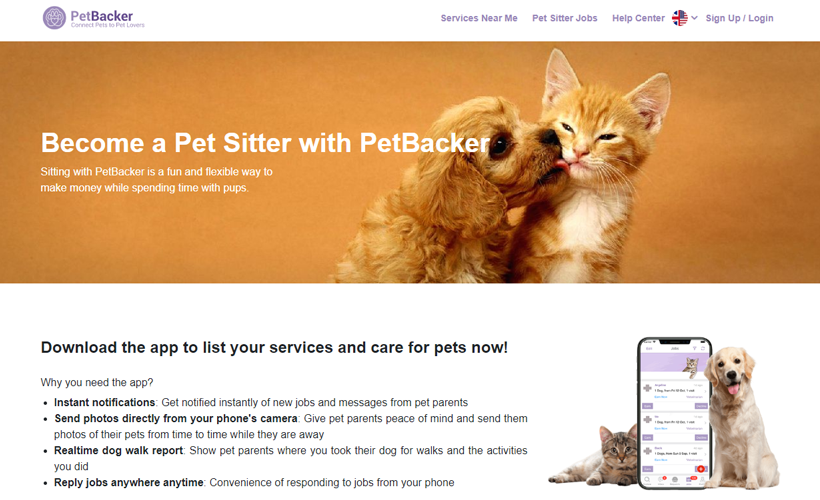This is a detailed screenshot from the Pet Backer website. In the main section, there's a charming image of an orange ginger cat and dog, sitting side by side and exuding friendliness as the dog affectionately licks the cat’s face. Below this heartwarming scene, a prompt encourages users to download the Pet Backer app, highlighting its features such as instant notifications, real-time dog walking reports, the ability to respond to jobs from anywhere, and tracking pet locations while under pet sitters' care. Additionally, the screenshot displays an image of a smartphone next to the cat and dog, emphasizing the app's user-friendly interface. The website's predominantly white design is accentuated with an orange central border.